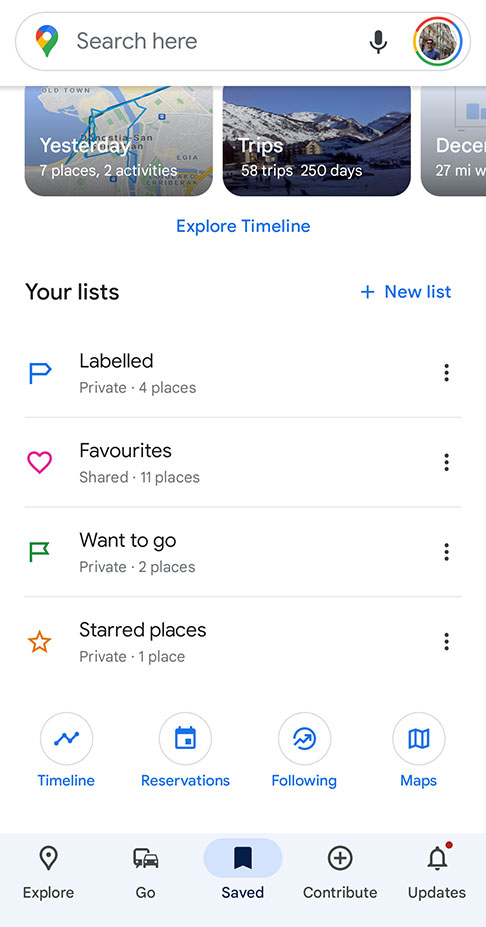The image depicts a mobile webpage interface designed by Google. At the top of the screen, there is a Google logo adjacent to a search bar that prompts users to "search here," accompanied by a microphone icon for voice search capability. To the right of the search bar, a user avatar is visible, indicating the current user's profile.

Below this header, there is a map graphic with a label indicating a mountain trip that took place yesterday, denoted as "December." A prominent blue button labeled "Explore Timeline" is displayed beneath the map. Further down, a section titled "Your List" outlines various categories: "Favorites," "Labeled," "Want to Go," and "Starred Places." These categories are accompanied by respective counts: 11 places in "Favorites" (which is shared), four in "Labeled" (private), two in "Want to Go" (private), and one in "Starred Places" (private).

Additional navigation options are listed with corresponding icons: "Timeline," "Reservations," "Following," and "Maps." At the bottom of the screen, there is a horizontal menu featuring five buttons: "Explore," "Go," "Save," "Contribute," and "Updates." The font and iconography throughout the interface maintain a consistent style and size, enhancing user experience and readability.